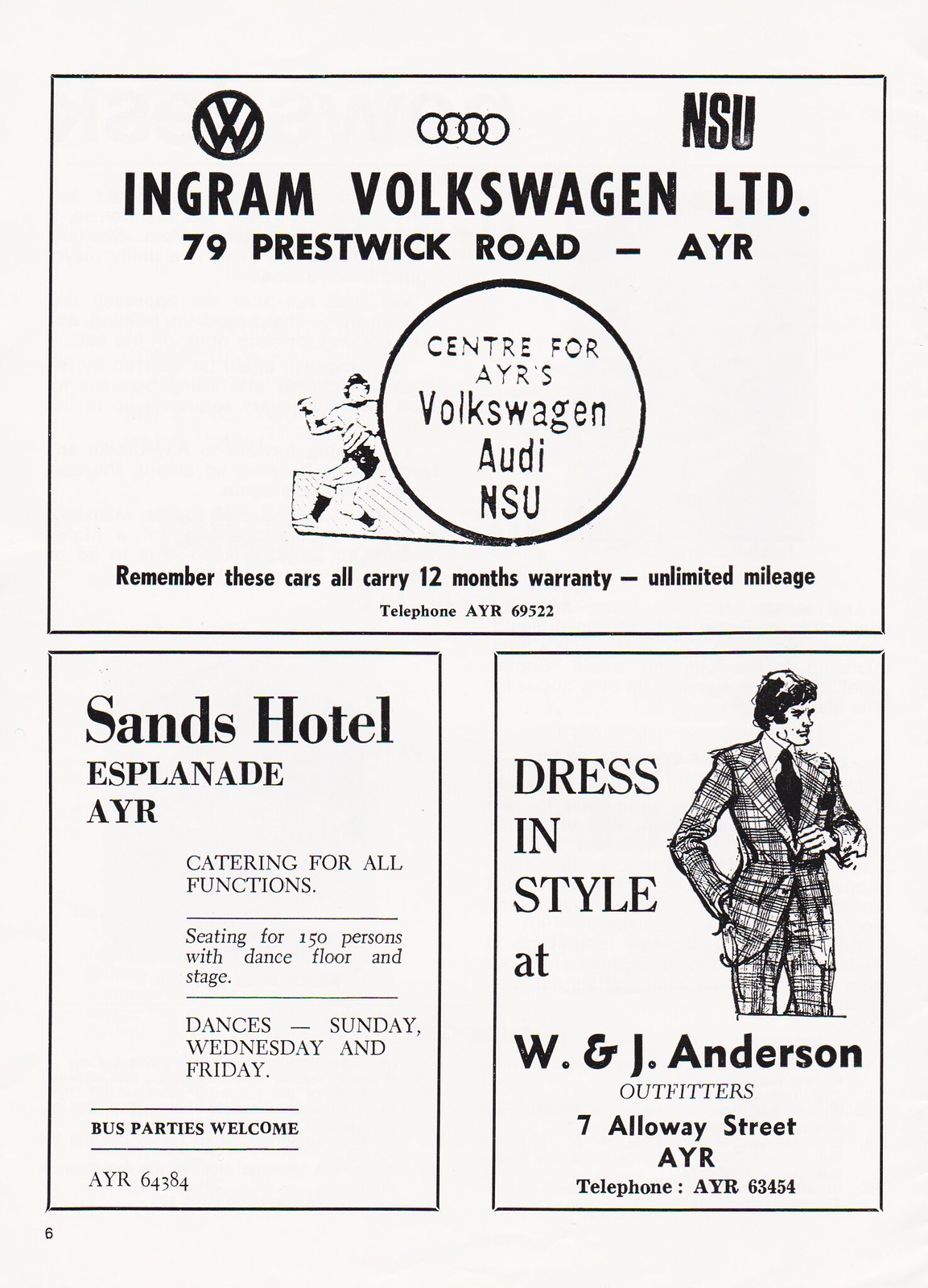The vertical rectangular image appears to be an old program page from a sporting event, featuring a collection of advertisements in black and white. The top half of the page is dominated by a large rectangular ad for Ingram Volkswagen Limited, with text prominently displaying the company name and address: "Ingram Volkswagen Limited, 79 Prestwick Road, AYR." Just below the company name, inside a conspicuous circle, are details about the cars sold, highlighting "Center for Ayr's Volkswagen, Audi, NSU." The ad further emphasizes that these vehicles come with a "12 months warranty, unlimited mileage," and provides the contact number "Telephone AYR 69522." A drawing possibly depicting a man or a soccer player is situated near the circle.

The bottom half of the page is split into two equal-sized rectangles side by side. The left rectangle advertises the Sands Hotel, located at "Esplanade AYR," offering "catering for all functions" with "seating for 150 persons with dance floor and stage." They host dances on "Sunday, Wednesday, and Friday" and welcome "bus parties," with the contact number "AYR 64384" provided. The right rectangle showcases a drawing of a man in a plaid suit and black tie, accompanied by text that reads, "Dress in style at W. & J. Anderson Outfitters, 7 Alloway Street, AYR," along with the telephone number "AYR 63454."

Overall, the page depicts a nostalgic snapshot of local businesses, encapsulated through carefully detailed advertisements.